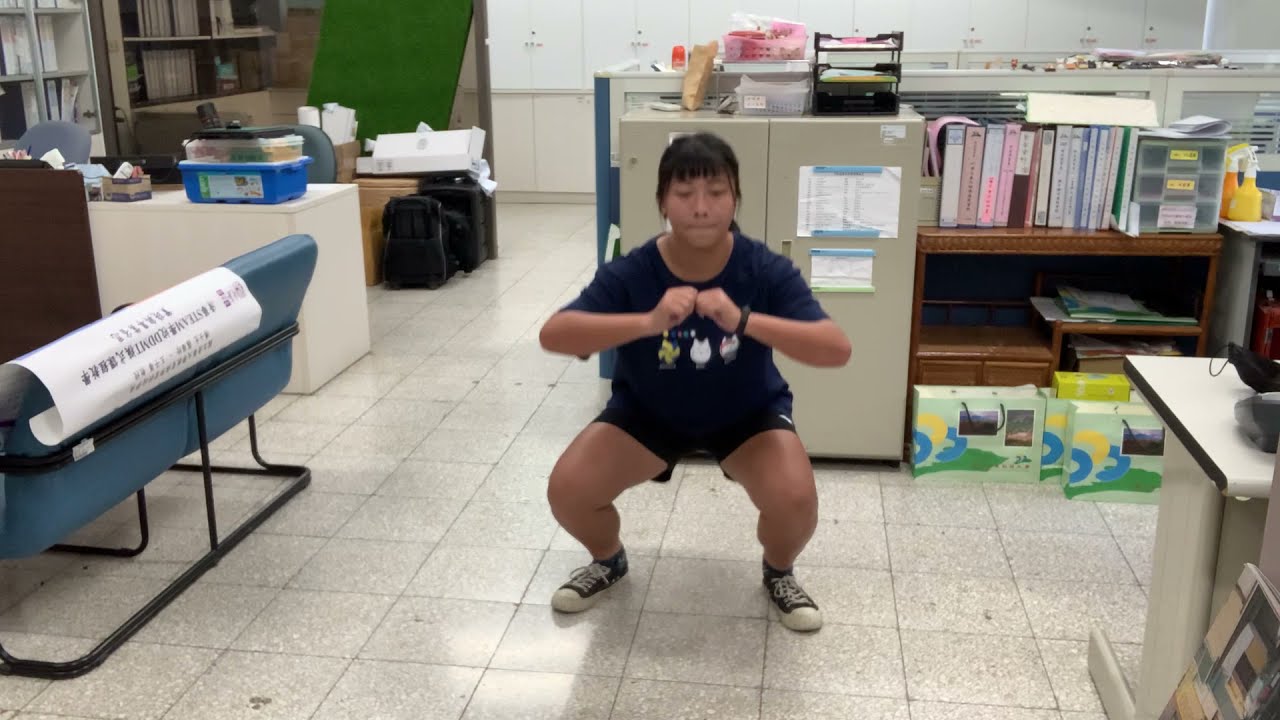The photograph depicts a young Asian girl with short black hair performing a bodyweight squat in the middle of a cluttered office or file room. She is facing the camera with a determined expression, her arms extended in front with fists together. Dressed in a dark blue t-shirt with printed icons and black shorts, she completes the outfit with black and white basketball-style sneakers. The room is characterized by a speckled off-white tile floor, surrounded by various office furnishings and clutter. To the left, there are several file cabinets, desks, chairs, a metal and blue sofa topped by a large white poster with black Chinese characters, and shelving units with files and paperwork. Behind her, there's a closed light grey metal filing cabinet with paperwork attached to it, and further back, white cabinets over a beige wall. On the right, more bookshelves and cabinets with binders and boxes can be seen. The overall space appears densely packed with books, boxes, and various office supplies.